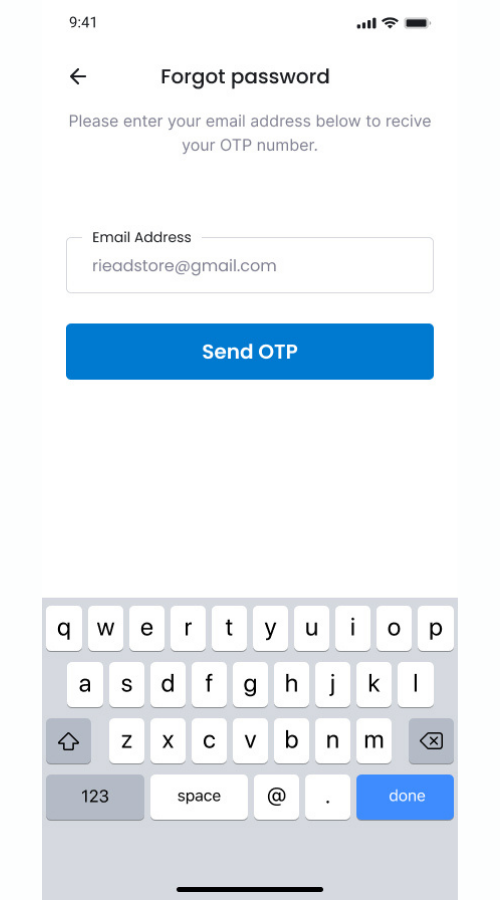A smartphone screenshot displaying the "Forgot Password" page. The time in the upper left corner reads 9:41, and the status indicators on the upper right show four bars of cell phone signal, active Wi-Fi, and a fully charged battery. Centered at the top is the title "Forgot Password" accompanied by a left-pointing arrow icon. Below, there is a prompt instructing the user to enter their email address to receive an OTP number. The email address "ryeadstore@gmail.com" is already filled into the input box. Beneath the input box, a blue button labeled "Send OTP" is prominently displayed. The lower part of the screenshot shows the smartphone's keyboard over a gray background.